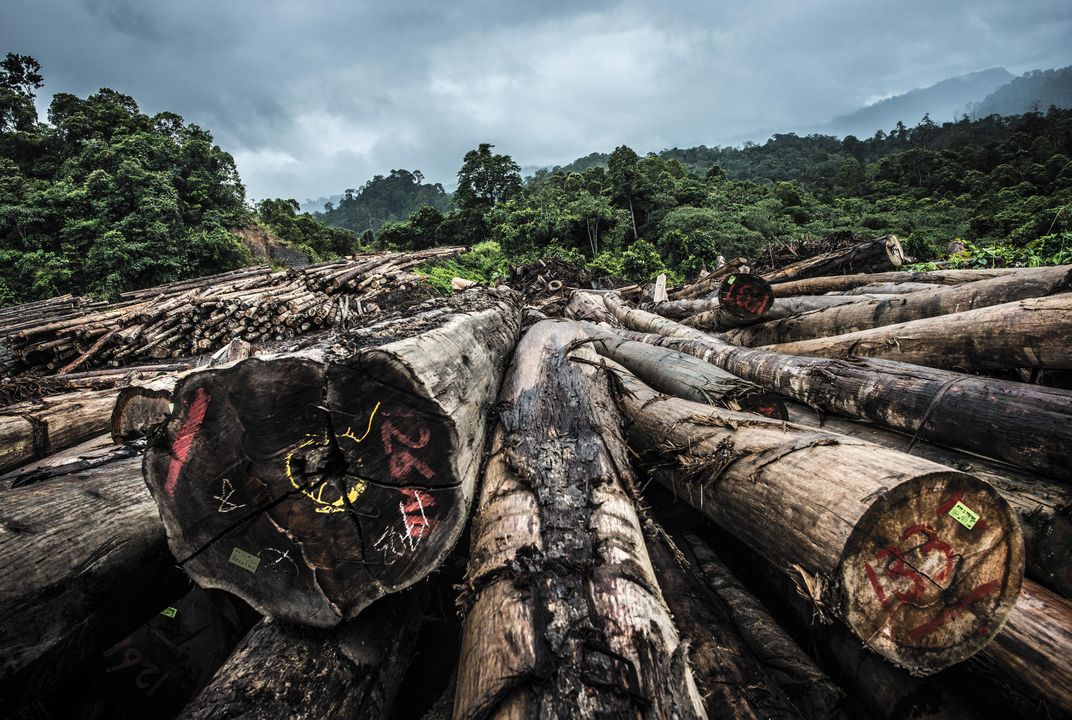The image depicts a stormy, overcast day with a gunmetal gray sky occupying about one-fifth of the horizontal frame. In the background, lush, dark green trees form a dense forest, and the upper right corner reveals a glimpse of distant mountains. The foreground dominates the scene with a chaotic yet organized arrangement of logs, their ends facing the viewer. The logs vary in color from gray and beige to darker hues, and several feature spray-painted markings, including red and orange numbers as well as distinct marks like "26A" in pink and a yellow circle. The bark on some logs appears peeled off, hinting at their raw state, presumably ready for shipment. The layered stacks of logs fan out and extend towards the camera, providing an intricate, detailed texture against the darker, moody atmosphere of the forest backdrop.